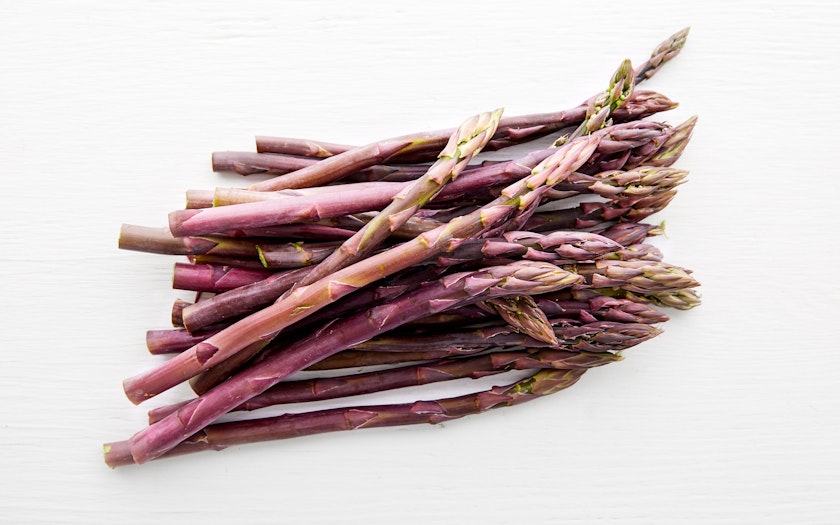The image features a striking pile of thick, purple asparagus with varying hues of pale pink, peach, and a touch of green, arranged against a bright white background with subtle ridges, possibly a faux wood surface. Approximately 20 neatly stacked spears lie horizontally, with their verdant tips pointing towards the right and the thicker bases clustered to the left. The asparagus spears exhibit a healthy, fresh appearance and retain their characteristic prickly textures. The lighting, sourced from the top and slightly above the upper right corner, uniformly illuminates the scene, casting minimal shadows, thereby highlighting the unusual color and intact nature of the asparagus.